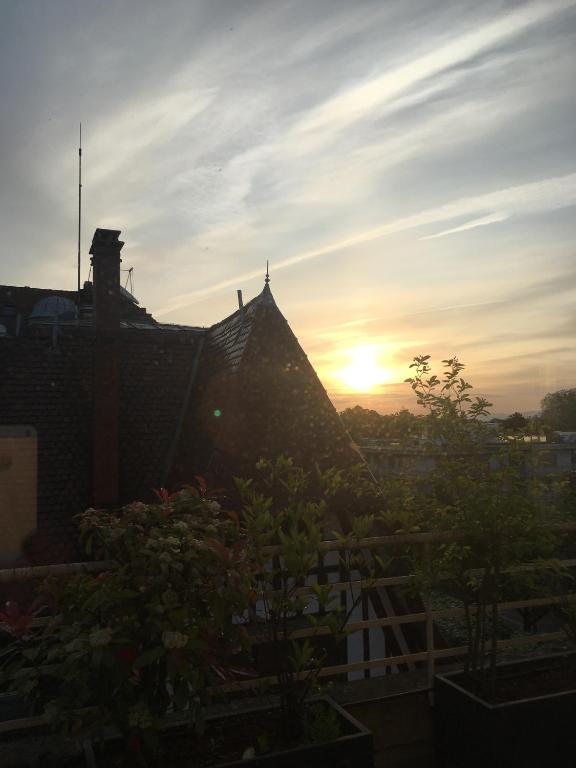The photograph captures a house in deep shadow against a vibrant, pastel-toned sunset. The sky, filled with streaky, light grayish clouds, adds to the ambiance of the setting sun on the horizon. The house, which appears to have white panels with dark wooden accents, features a chimney with a visible antenna. To the right of the house, a large green tree stretches towards the roofline, and to the left, the silhouette of another house is partially visible. The scene has a distinctly Dutch architectural feel. Below and in front of the house lies a garden filled with various plants and flowering bushes, their forms silhouetted against the dimming light. Adding depth to the scene, a wooden fence with clearly defined horizontal lines runs across the foreground. The overall image is characterized by darkened, intricate shadows, giving a moody yet picturesque depiction of the serene setting.